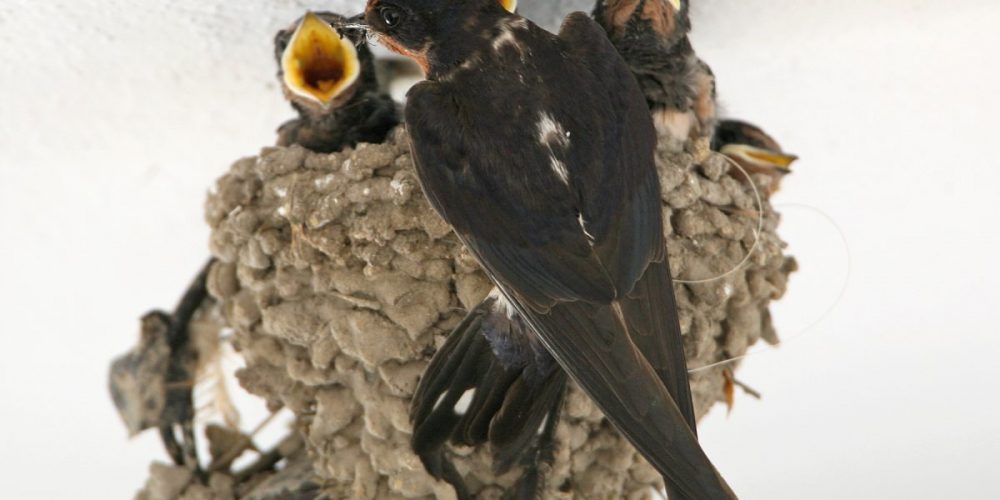The image is a horizontally oriented photograph featuring a central scene of birds. Dominating the foreground is a dark brown bird with some white marking down its back and an orange patch under its beak, appearing to face away from the camera. This bird has debris in its beak and appears to be perched on a nest-like structure, possibly composed of mud or dirt. The background is a light gray. There are two brown, cloth-like objects hanging down to the right side of the central bird. 

Near the central bird, there seems to be several younger birds in varying conditions. One bird, likely deceased, lies on its back with its beak wide open, showing a yellow interior. This bird seems to be trapped under a honeycomb-like structure. There's another bird with its beak open and tongue visible, perhaps being fed by the mother bird. Just to the left of the brown cloth objects is a distinct flower with a yellow center and darker brown details, along with a glass-like eye below it, contributing to the complex tableau of the image.